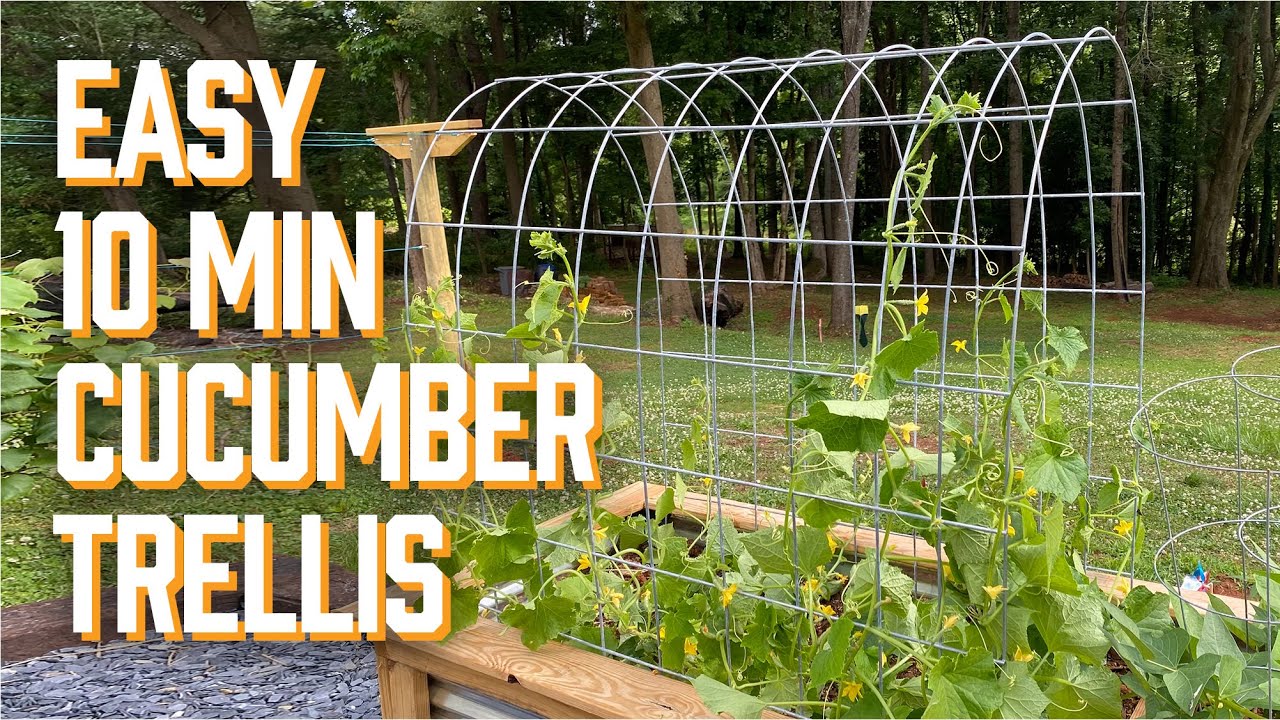The vibrant outdoor photograph showcases a well-maintained backyard garden scene. On the left side of the image, bold text reads "Easy 10 Minute Cucumber Trellis," suggesting the photograph is a thumbnail for a YouTube video, blog, or advertisement. The right side of the image features a wire-arched trellis set within a long, square wooden garden bed elevated off the ground. Cucumber vines, adorned with yellow blossoms, climb the trellis and sprout from the soil in the garden bed. The bed is placed in a meticulously manicured grassy area, framed by lush, full-grown trees that add a sense of tranquility to the scene. Small stones decorate the garden area, contributing to the garden's aesthetic appeal. The bright sunlight illuminates the greenery, making the predominant color of the image a vivid green. This detailed image serves as a visual guide for creating and utilizing cucumber trellises for healthy cucumber growth in a home garden setting.